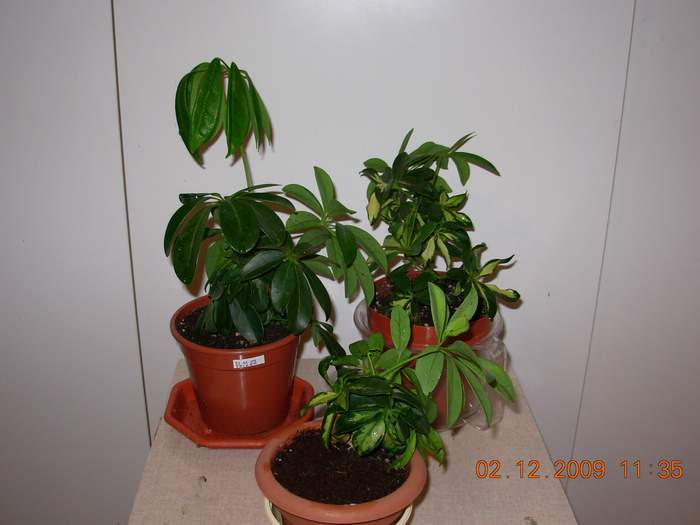This detailed and vibrant image, taken on February 12, 2009, at 11:35 p.m., captures three potted plants sitting atop a small, square coffee table. The background is a white wooden panel wall divided into three sections, perhaps part of a wardrobe. The bottom right-hand corner of the image displays the date and time watermark, indicating that the photograph was taken with a digital camera, possibly with a flash, given the noticeable shadows.

The potted plants each have their own unique attributes. On the left side, a light brown clay pot is filled with a lush assortment of green foliage. The middle pot, a reddish-brown hue, contains a single flower that appears slightly bent out of shape. On the right side, another pot, similar in color to the one in the middle, houses a plant with a variety of green shades, creating a dynamic and vibrant scene. The interplay of light and shadows emphasizes the vividness of the leafy greens, making the plants stand out against the stark white background.